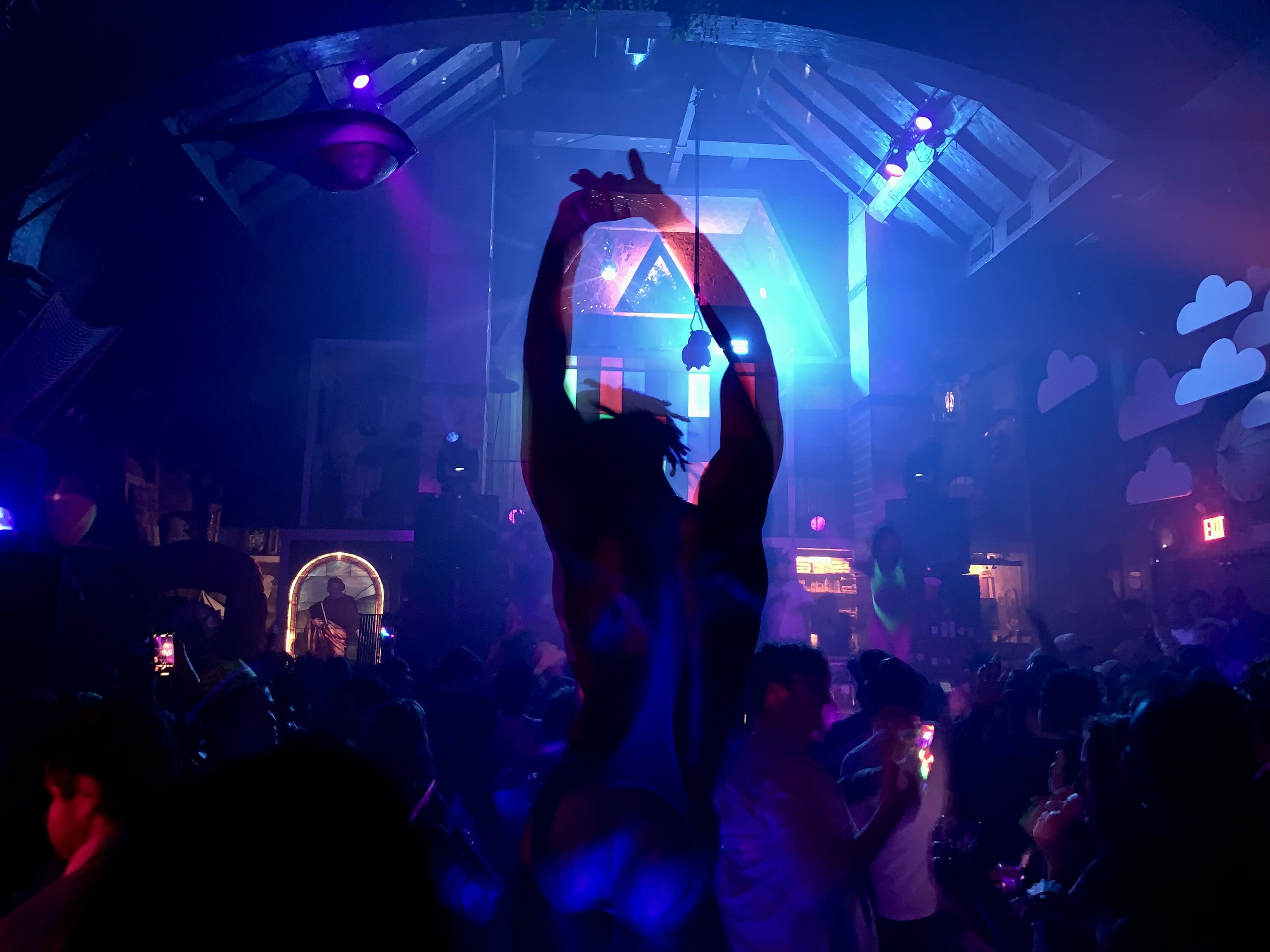In the dimly lit scene, a muscular man with dreadlocks stands center stage, silhouetted against a backdrop of ethereal purple and blue hues, with his arms raised and fingers clasped above his head. The setting evokes a lively dance club atmosphere, suggested by the spotlights casting colorful lights and the faint outlines of other partygoers surrounding him. From the ceiling, lights beam down, casting a mix of light purple, blue, and red tones that enhance the shadowy, almost cinematic feel of the scene. To the right, there are whimsical, cloud-shaped cutouts decorating the wall, adding to the surreal ambiance. In the lower left, a stained glass window peeks into view, hinting at the venue's possible past as a church. The entire visual is enveloped in a dark, mysterious palette, making it challenging to determine the specifics but vividly capturing the essence of an energetic concert or dance party.